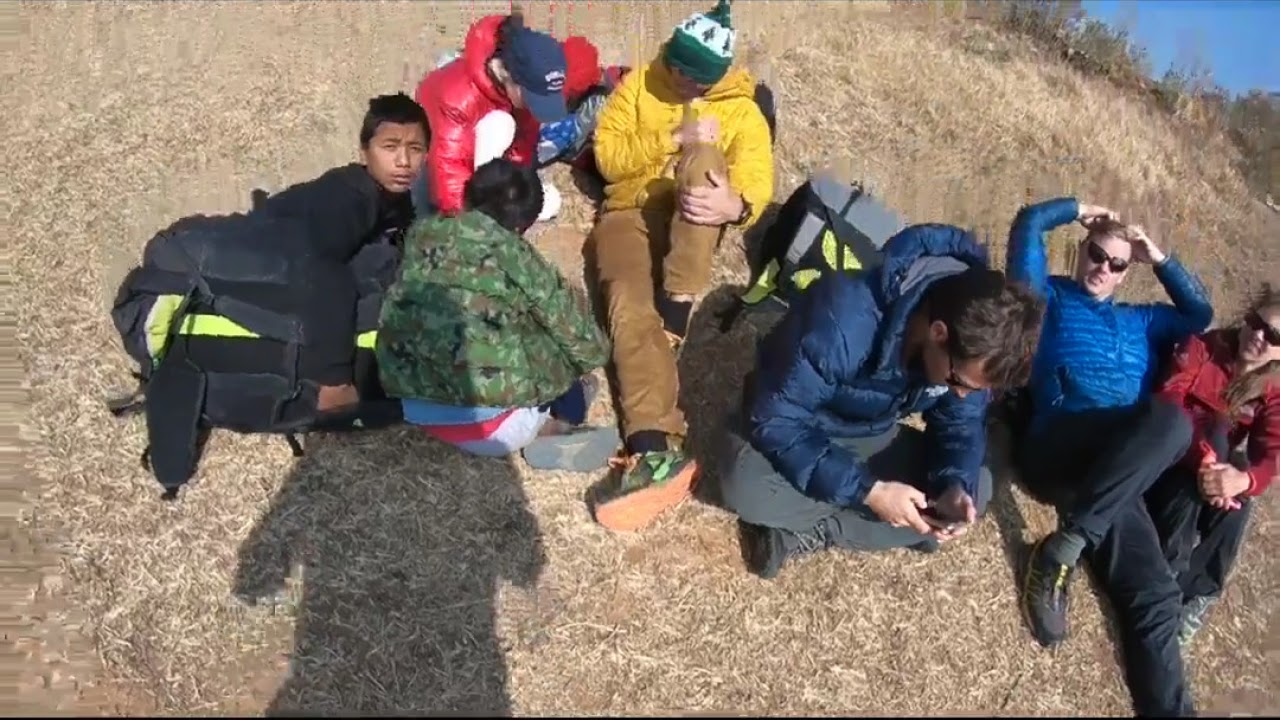This image captures a group of seven hikers resting on a grassy slope under a clear sky. The slope ascends from the bottom to the top of the frame, creating a dynamic composition. The person on the far left is a brown-skinned individual dressed entirely in black, accented by a yellow waist belt. Next to him, a man with his back turned to the camera is wearing a green camouflage jacket layered over a gray and red shirt, paired with whitish-gray pants. Above him, another man in a thick red jacket and white pants is glancing downward to his right. Beside him, a man is seated with his right leg extended and his hands holding his bent left leg, wearing a green and white beanie, yellow jacket, and brown pants. Further to the right, a man in a thick blue shirt and gray pants also looks downward. Continuing to the right, a relaxed man leans back with his hands behind his head, smirking at the camera under his sunglasses, dressed in a light blue jacket and dark black pants. The woman on the far right sits with her knees drawn up and her hands clasped around them, wearing a red jacket and black pants. Shadows, including that of the person taking the picture, fall across the ground, adding depth to the scene. The group, equipped with backpacks and heavy winter clothing, likely suggests a cold, mountainous environment, possibly high in altitude.